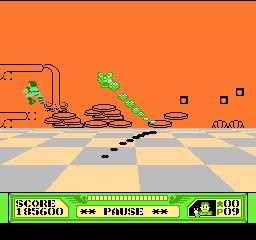The image is a screenshot of what appears to be a vintage or retro-styled video game. The top half of the screen features a bright orange background with black coin-like shapes scattered in the distance. The central portion of the screen displays a tannish and light blue checkerboard floor that seems to round off toward the top. There are little green characters casting shadows as they fly up in the air amidst these coins. At the bottom of the screen, a green rectangle holds the game interface: the score of 185,600 on the left, the word "PAUSE" in capital letters in the center, flanked by two asterisks on each side, and the player's statistics on the right, including a small character icon beside the numbers "00" and "P09" along with a star icon. Completing the screen, a black bar stretches across the very bottom, filling the remaining space and providing a clean separation from the game interface above.